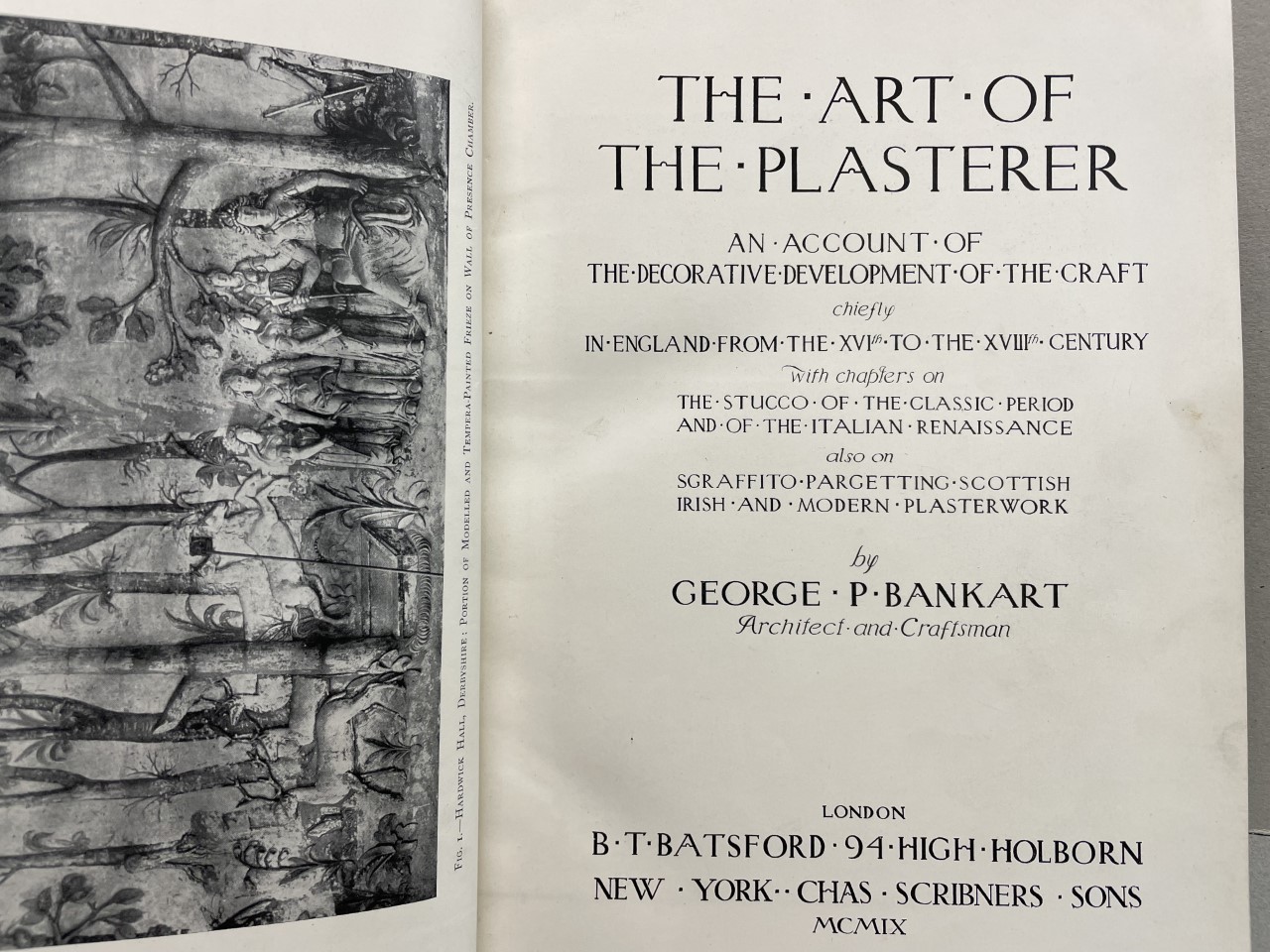The image is a detailed photograph taken indoors depicting the inside of an open book. The book is rectangular, approximately six inches wide and four inches high. On the left page, there is a black and white drawing that appears to be a photograph of a carving. The carving depicts a scene in the woods with people, deer, and possibly cows, surrounded by trees. There's text along the border of the image, but it is too small to be legible.

The right page features the book's title and additional information in bold and smaller print. At the top, it reads "The Art of the Plasterer." Below that, in smaller text, it states "An Account of the Decorative Development of the Craft chiefly in England from the 16th to the 18th Centuries, with chapters on the stucco of the classic period and of the Italian Renaissance. Also on sgraffito, pargetting, Scottish, Irish and modern plaster work by George P. Bankart, architect and craftsman." At the bottom, it mentions the publication details: "London, BT Batsford, 94 High Holborn. New York, Charles Scribner’s Sons."